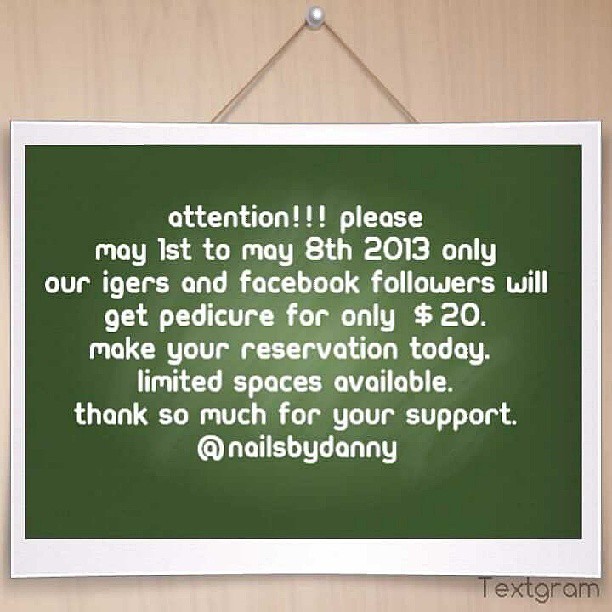This image showcases a green digital board with a gradient effect, hanging on a platform wall, fastened with a pin and yarn at the top. The board is encircled by a white and gray border and has a faux woodgrain pale tan backdrop. Displayed in bold, white lowercase letters, the notice reads: "Attention! Please, May 1st to May 8th, 2013, only our IGs and Facebook followers will get pedicure for only $20. Make your reservation today. Limited space is available. Thank you so much for your support. At Nails by Danny." There is clear punctuation throughout the text. In the bottom right corner of the board, the word "Textgram" indicates the app used to create this design.